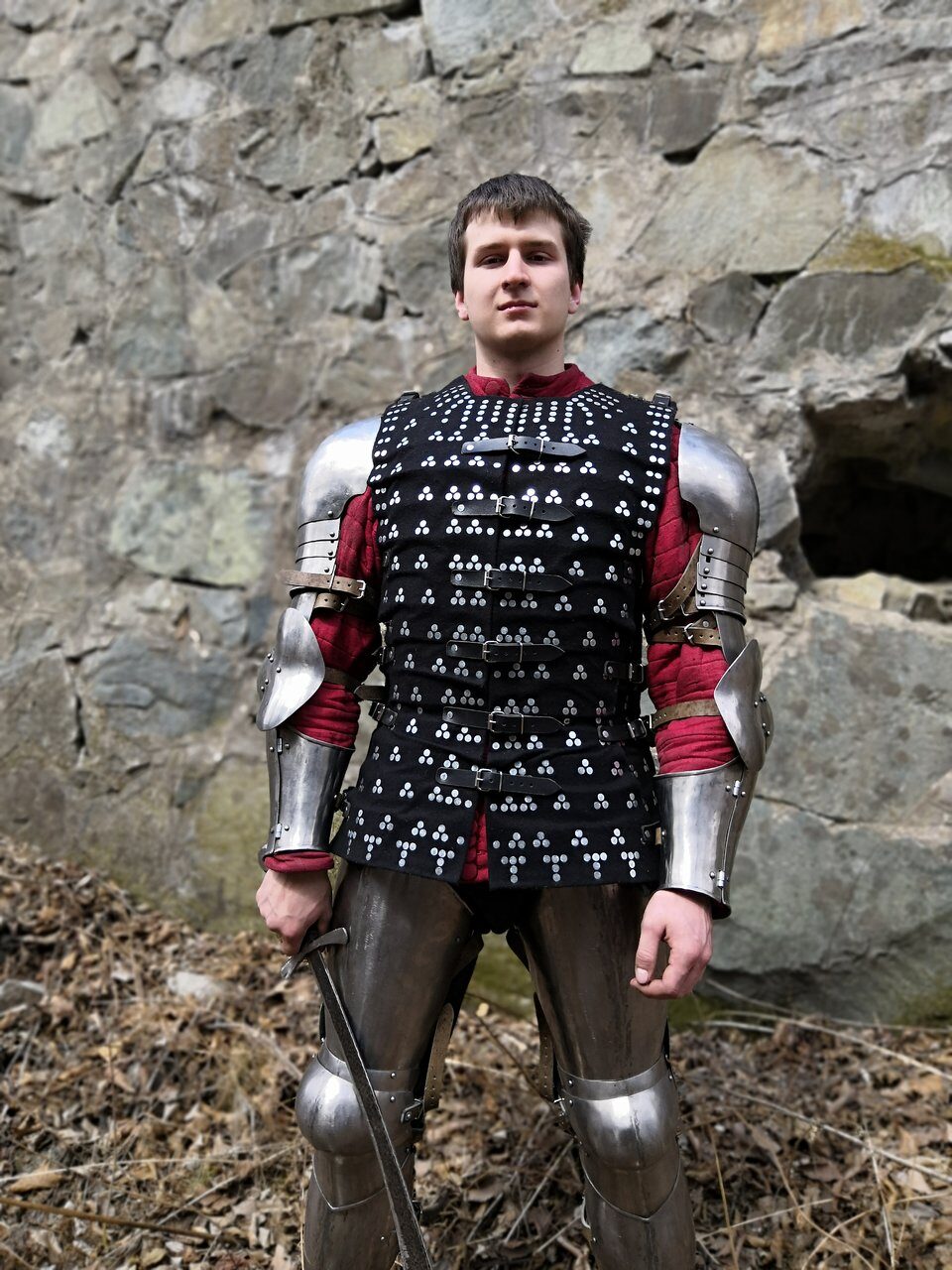The image features a young man, estimated to be between 15 to 25 years old, standing confidently in front of a large rock structure. The ground is littered with dead leaves and sparse grass. The man has short brown hair with visible bangs above his eyes and is clad in an elaborate knight's uniform. His attire includes a shiny, red puffy undershirt, and over it, he wears substantial metal armor. The armor consists of silver shoulder pads, elbow pads, and bracers on his arms, as well as matching metal armor pieces on his legs. His chest is protected by a distinct large black chest plate, adorned with multiple triangularly arranged dot patterns and fastened by several buckle straps. In his right hand, he holds a sleek metal sword, while he gazes smugly at the camera.